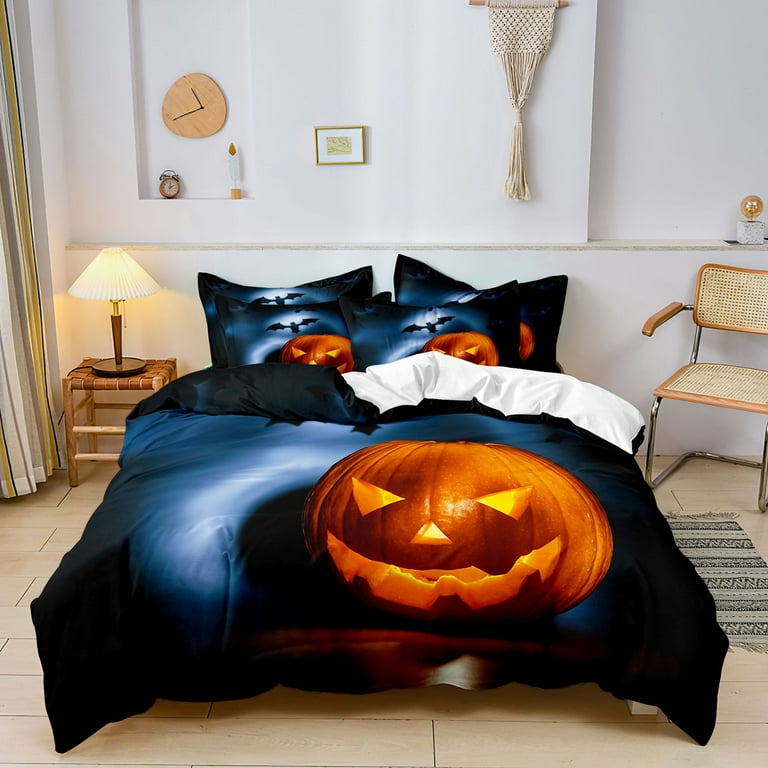This photograph captures a cozy, Halloween-themed bedroom decorated in an off-white and light beige color palette. The centerpiece is a bed adorned with a dark blue-black bedspread featuring an orange, grinning jack-o'-lantern with triangle eyes and nose under a bat-flying cloudy sky, perfectly coordinated with matching pillows. The floor is a light beige color and to the left of the bed stands a small wooden nightstand holding a lit lamp that casts a warm yellow glow. On the right side of the room, a chair is situated with a gray and beige striped rug in front of it. Above the bed, there is a macrame wall hanging, an abstract clock, and a small picture frame, adding an artistic touch to the space. The overall ambiance is both festive and inviting, with elements that give the impression of the jack-o'-lantern almost popping out in 3D.